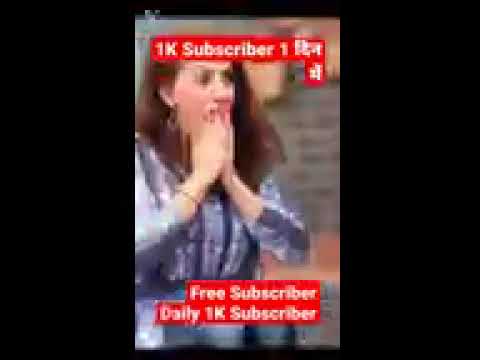This image appears to be a grainy screenshot of a social media reel, possibly from TikTok, designed as an advertisement. The primary focus is a white woman, seemingly in her 30s or early 40s, who has shoulder-length brown hair. She wears a blue, striped blouse with a possible floral print. Her mouth is agape in a perfect 'O' shape, and she holds her hands, with fists clenched, just above her shoulders, expressing surprise or astonishment.

The image is colorized in the center but has a black-and-white, zoomed-in, and faded background featuring a close-up of her face. Overlaying the image are red banners with white text: at the top, "1K subscriber" and at the bottom, "free subscriber, daily 1K subscriber." This text suggests the advertisement promotes a service that offers daily subscribers, possibly to inflate social media followings artificially. The pixelated and slightly low-resolution visual gives it an authenticity, as if captured from a smartphone such as an iPhone or Android.